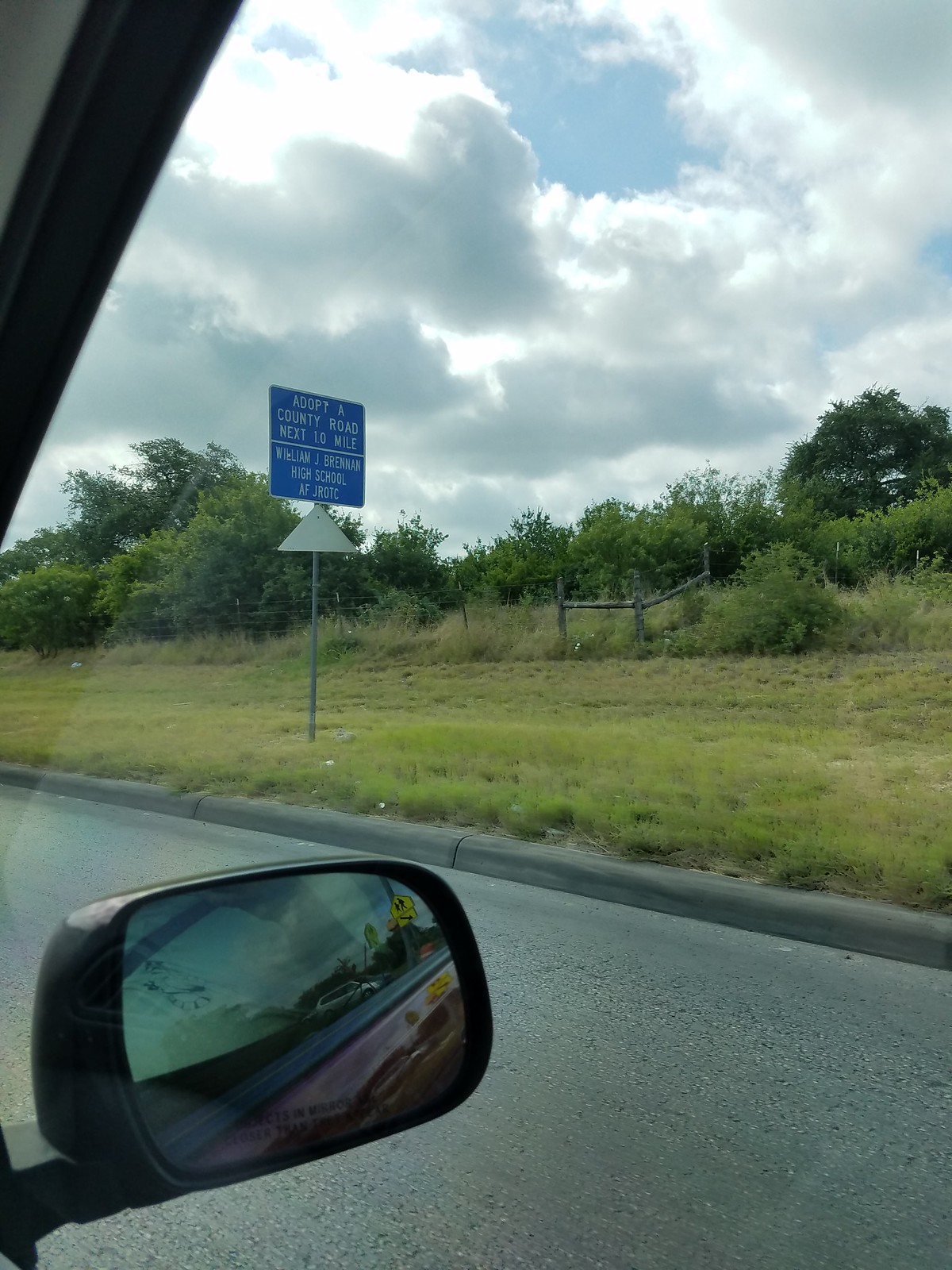The photograph captures a scene from inside a car, focusing through the window on the left side of the vehicle. The edge of the car window is visible along with the car’s side mirror, which reflects the car's window and door, adding depth to the image. Outside, the scene reveals a gray, paved road bordered by a curb, with an adjacent grassy area that is a muted green in color. Prominently, there is a white sign by the curb which reads “Adopt A County Road Next 1 Mile, William J. Brennan High School, AFJROTC,” emphasizing community involvement in maintaining the area. Beneath this sign, another smaller triangular white sign is visible but unreadable. The background features a line of trees under a cloudy, overcast sky, giving the photograph a subdued, tranquil atmosphere.